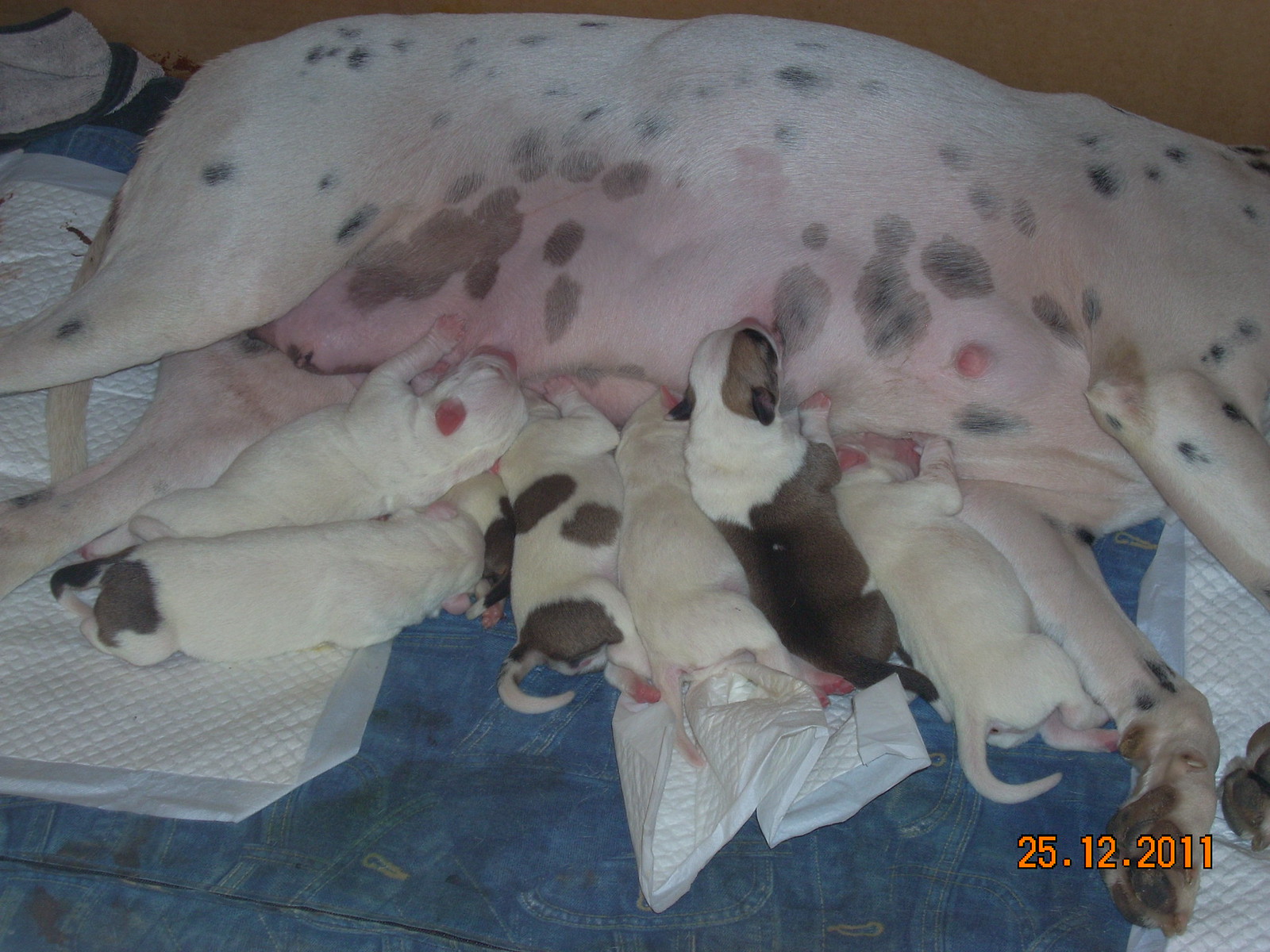The image, time-stamped 25th December 2011, vividly captures a tender moment between a mother dog and her newborn puppies, likely only a day or two old. The mother, with a coat of thick, Dalmatian-like spots, is lying on her side on a blue denim surface, cushioned by absorbent pads around. Her head is out of the frame, but her legs stretch out, providing a nurturing presence to her litter. There are seven puppies in total: three are entirely white, one is predominantly white with a blackish-brown spot on its rump and tail, and three exhibit large, distinct spots with varying patterns. One puppy is notably resting on top of a sibling. All the puppies are nursing contentedly, some looking so full that they're already falling asleep. This photograph captures the serene and nurturing atmosphere of a mother and her pups on their first Christmas, reflecting the pure joy and peace of new life.